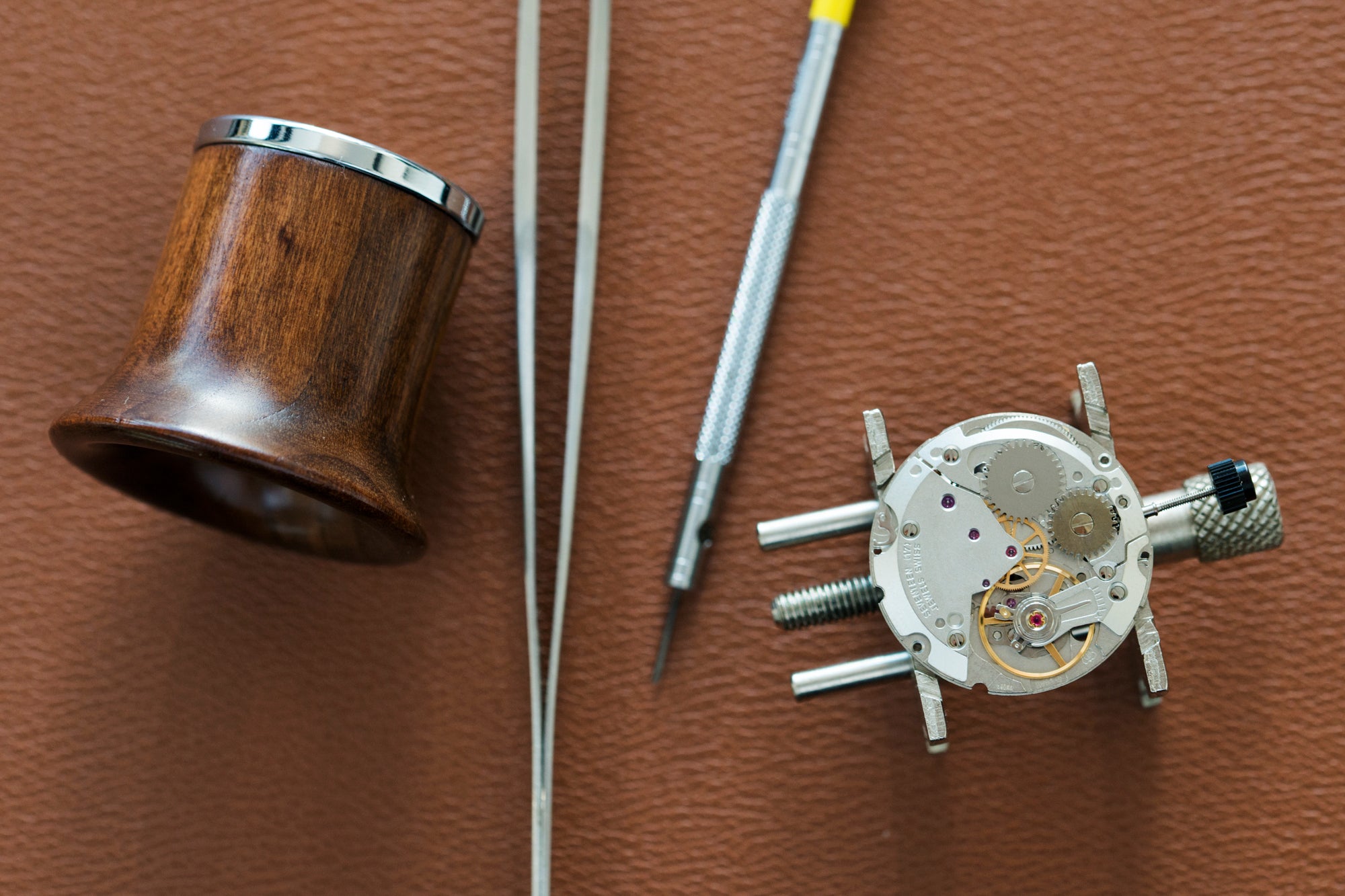In this top-down photograph, four distinct objects are arranged on a brown backdrop, which appears to be a leather surface. On the left, there is a cylindrical wooden structure with a flared bottom and a silver metal band near the top. The next object, situated to its right, resembles a pair of silver tweezers with a narrowing tip, though the base is obscured. The third item is a slender, silver precision screwdriver with a yellow top and a screw-like bottom. Finally, on the far right, there is a complex mechanical component, possibly a watch part, featuring a central gear-like mechanism with four extensions and a metal post projecting from its right side. Additionally, there are three screws emerging from the left side of this gear, indicating it is likely part of a larger device.